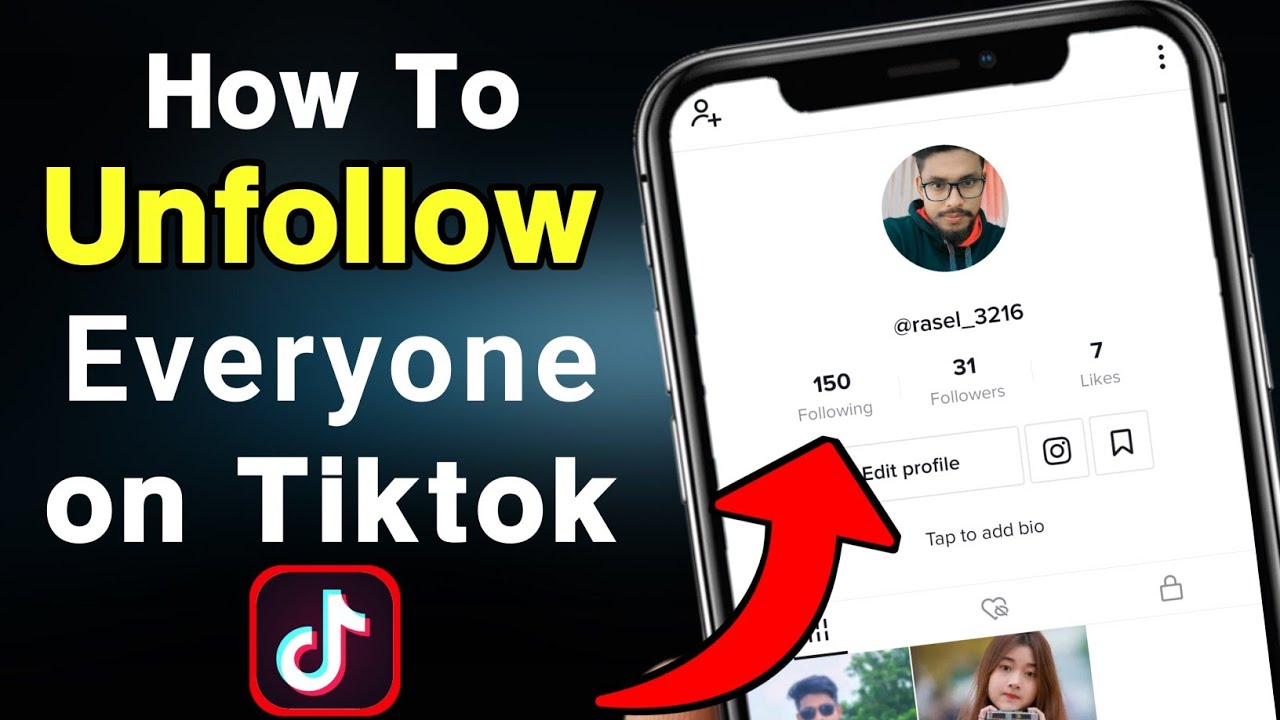In this advertising image, a sleek, silver mobile device resembling an iPhone is prominently displayed. The device features a visible speaker and camera at the top. The screen of the device shows a TikTok profile, highlighted against a white background. 

The profile belongs to a man with dark hair, who is seen wearing glasses, a black sweatshirt, and sporting a goatee and mustache. The backdrop behind him is a mix of white and pink hues. 

On the profile interface, the profile button is situated to the far left, with the ad button nearby, and three vertical dots located in the upper right corner. A striking red arrow points to the user's stats, showing 150 following, 31 followers, and 7 likes. Below this, there are buttons labeled "Edit Profile," a camera button, and a save button.

A prompt "Tap to add bio" is visible under the profile name. The profile also includes two videos in the collection, symbolized by a gray lock button and a gray heart button. Large white text stretches across the screen, reading "How to" with the word "Unfollow" written in bright yellow. At the bottom of the image, "Everyone on TikTok" is displayed alongside the TikTok logo.